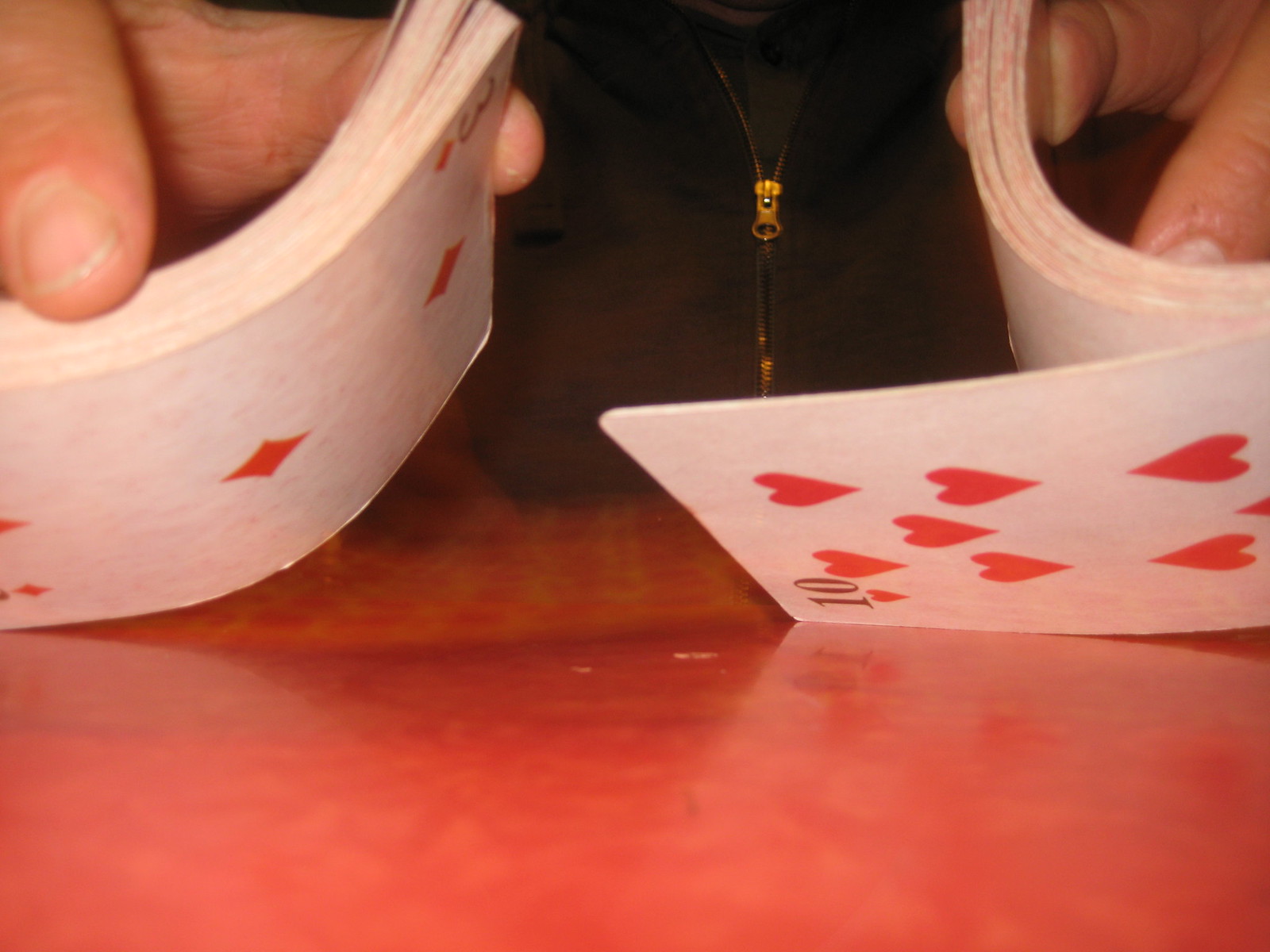In this detailed close-up image, we observe a person in the midst of shuffling a deck of cards. On both the left and right sides of the frame, stacks of cards are bent upwards, gripped firmly by the person's fingers. On the right stack, one card, the Ten of Hearts, has already been placed down on the table. On the left side, where the cards are arched, the next card to be dealt is visibly the Three of Diamonds. The person’s thumb and fingers are visibly holding and manipulating the deck with precision.

Dominating the central region of the image is the person’s shirt—a button-up sweater with a gold colored zipper that is halfway open. The surface beneath the action is a light red table with hints of orange, softly reflecting the shadows of the cards and the Ten of Hearts, which glimmers gently under the light. The person's fingernails are clearly groomed, displaying a natural pink hue with white tips.

Additionally, on the table’s surface, near the center, a small white speck—possibly a scratch—draws subtle attention amidst the meticulous card play. The reflections and shadows lend depth to the scene, highlighting the tension and anticipation of the card shuffle.